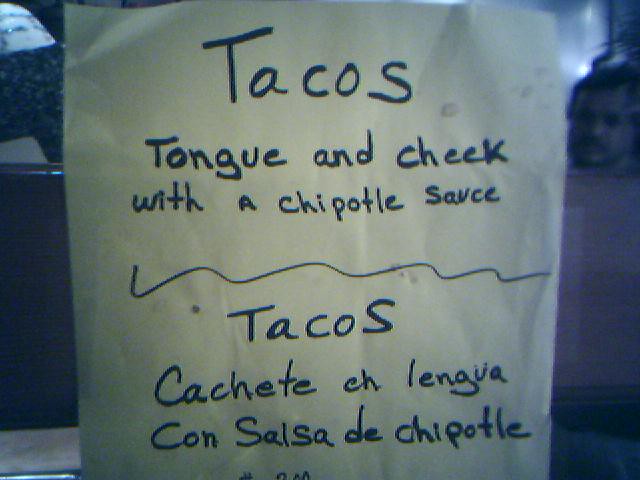In this image, there is a hand-drawn sign on a piece of white paper. At the top of the sign, written in black Sharpie marker, it reads "Tacos" with a capital 'T' followed by lowercase 'a-c-o-s'. Below this, in the same black marker, it states "tongue and cheek with a chipotle sauce", carefully written without any abbreviations. Separating the English text from the Spanish translation below is a squiggly line that extends from right to left. Underneath the squiggly line, the text continues in Spanish, reading "Tacos Cachete y Lengua Con Salsa de Chipotle", accurately spelled as "C-A-C-H-E-T-E E-L-E-N-G-U-A C-O-N S-A-L-S-A D-E C-H-I-P-O-T-L-E."